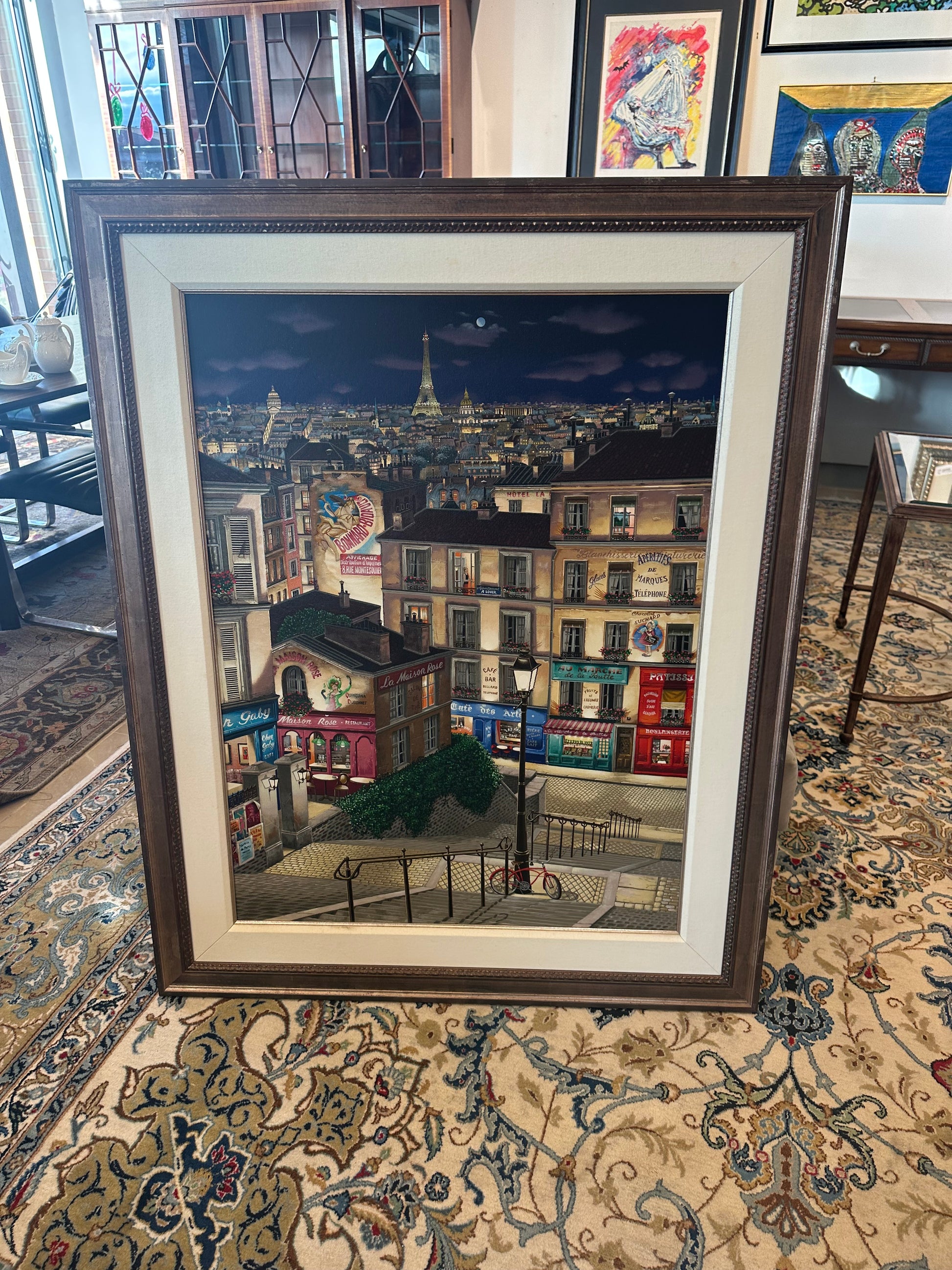The image captures a detailed scene of an opulent, well-lit room adorned with various pieces of art and luxurious furnishings. Dominating the foreground is a large, dark brown wooden picture frame resting on an ornate carpet. The carpet, featuring beige, blue, and maroon elements, adds a touch of elegance to the setting. The framed picture within this prominent frame showcases an overhead outdoor view of a large, vibrant city. The cityscape includes a busy courtyard area at the bottom, complete with buildings, a bicycle, and a lamppost, while in the background, a stunning skyline is visible, highlighted by the iconic Eiffel Tower and a moonlit sky.

In the room itself, which is brightly illuminated by indoor lighting that contrasts with the darker tones of the picture, there are several other picture frames mounted on the walls. To the upper left, a distinguished china cabinet stands, while the lower left features a small table accompanied by a chair. On the right side, one can observe additional wooden tables and more paintings, contributing to the room's refined ambiance. Overall, the room’s clarity and brightness, enhanced by natural light, create a striking setting for the vivid and detailed large picture frame, making it the focal point of this captivating visual composition.